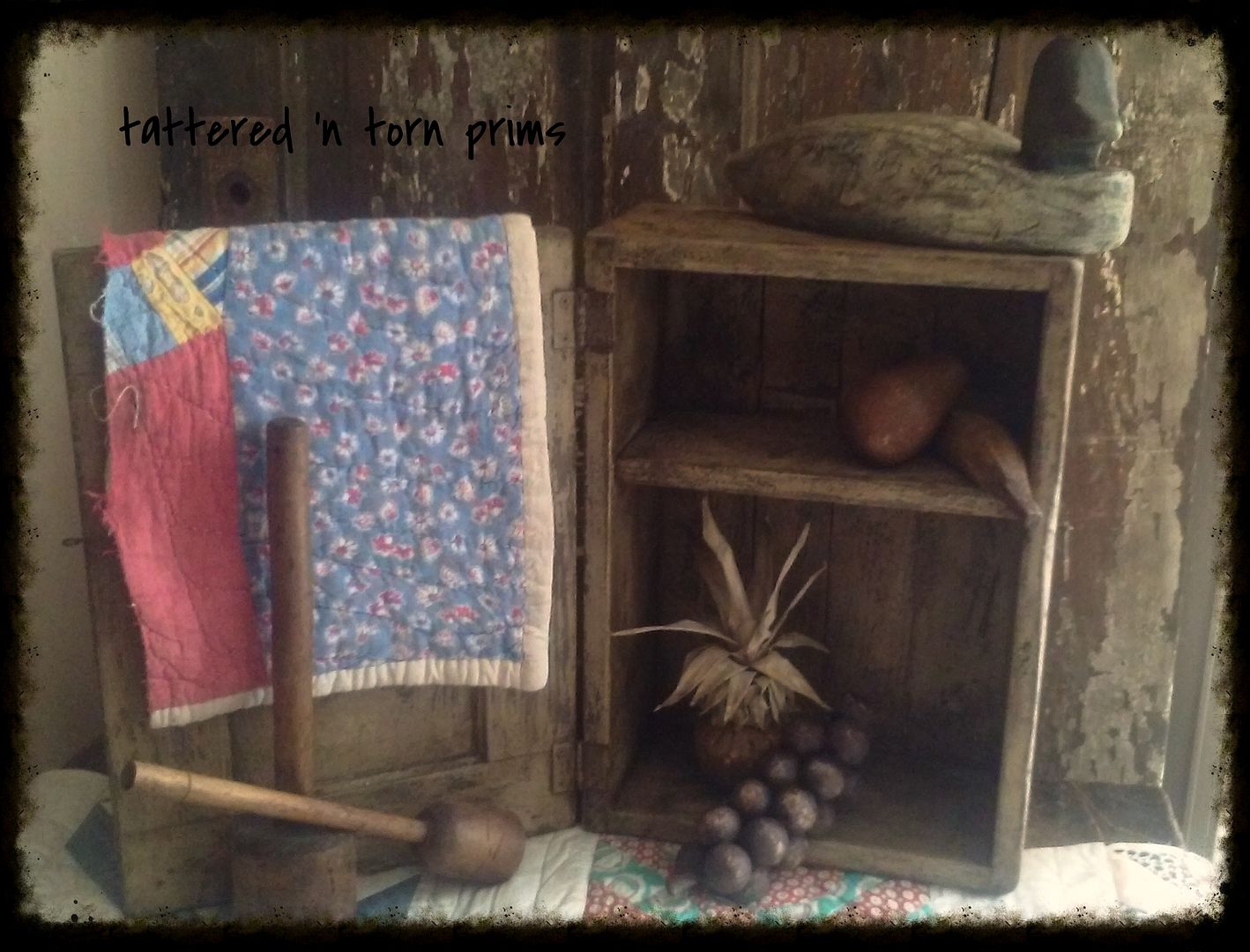The image features a rustic display from "Tattered and Torn Prims." Central to the scene is an open wooden chest divided into two storage cavities. Draped over its door is a handmade quilt with a floral design in yellow, blue, and pink, suggesting an unfinished piece. Inside the chest, the top shelf appears to hold carved wooden sweet potatoes, while the bottom shelf houses similar wooden carvings of grapes. Atop the chest sits a wooden duck, possibly a decoy. Several wooden tools, including a round mallet with a pole and a base, are arranged around the display, set against a background of a faded, rotting wooden wall. The entire arrangement rests on another quilt with a more professional finish, displaying circles that get progressively smaller inward. The image has a black digital vignette effect, and overlaid text includes "Tattered and Torn Prims" at the top, and "Photo Bucket" with the phrase "Protect more of your memories for less" towards the bottom.